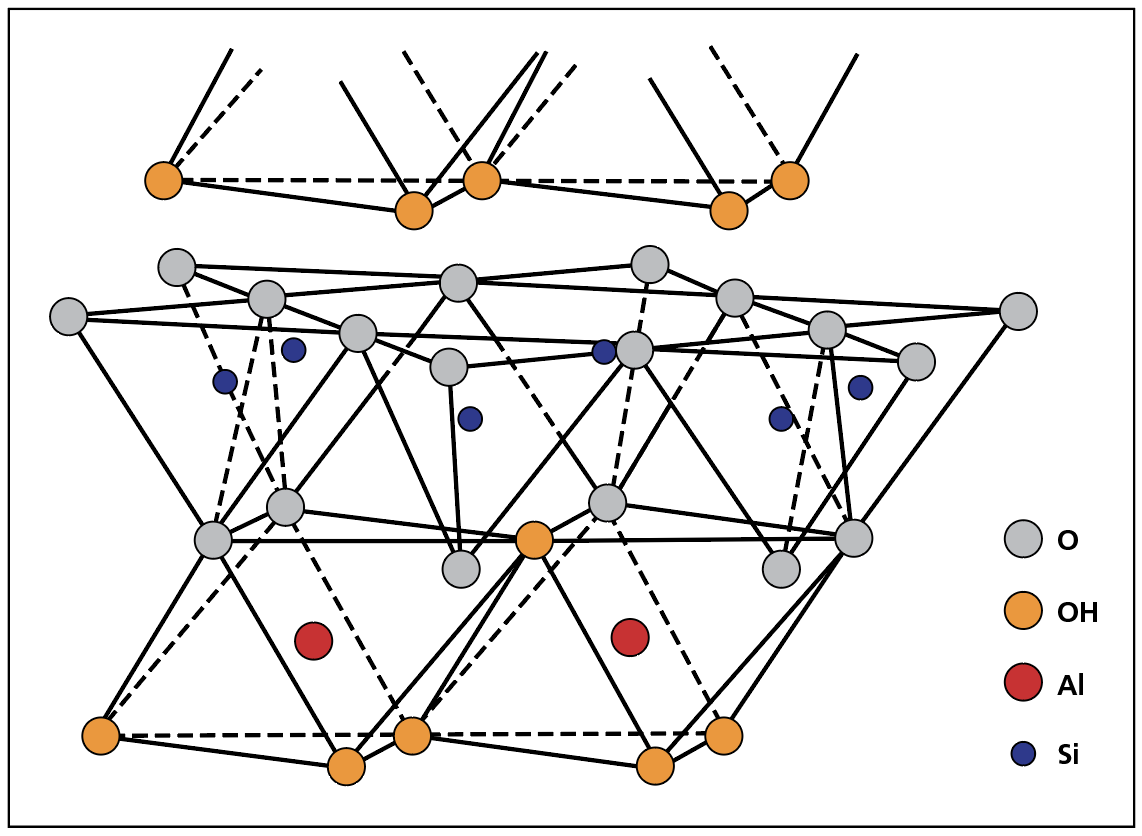The image features a detailed chemical diagram set against a white background, depicting a molecular structure through a series of interconnected circles and lines. The diagram includes both solid and dotted black lines, indicating different types of connections, such as covalent and hydrogen bonds. The circles come in various colors: light blue, dark blue, orange, red, and gray, each representing different atoms or groups within the molecule.

At the top of the diagram, larger light blue circles labeled 'O' (oxygen) are prominently displayed, often connected to smaller dark blue circles labeled 'Si' (silicon). The orange circles, labeled 'OH,' are distributed throughout the structure, signifying hydroxyl groups. Red circles, marked 'AL,' indicate aluminum atoms, and gray circles labeled 'O' also represent oxygen atoms, perhaps in different bonding contexts.

The molecular diagram is cohesively organized with each color-coded circle representing a different atomic element or functional group. This network of circles illustrates the complex connectivity within the molecule, providing a clear and colorful representation of the substance's chemical composition and spatial configuration.